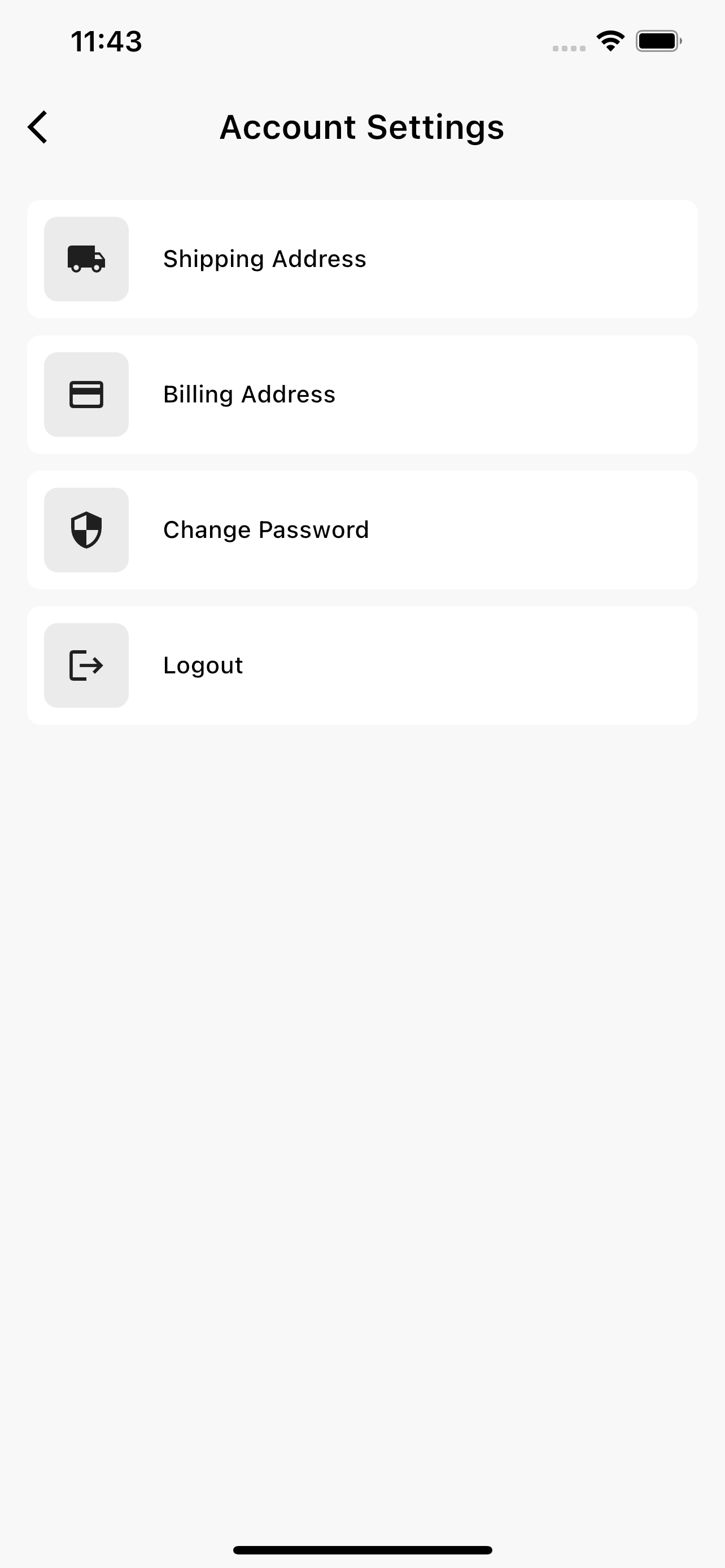The image presents a user interface on a gray background. In the top left corner, the time is displayed as 11:43. The top right corner features several icons: a series of four squares arranged side-by-side, a Wi-Fi signal indicator, and a full battery symbol. Below these icons, a left-facing chevron (less than symbol) is shown on the left, while the centered text reads "Account Settings."

Beneath this header, there are four white rectangular options:

1. The first has a gray box on the left with a truck icon, labeled "Shipping Address."
2. The second features a gray box with a grid or square-line icon, labeled "Billing Address."
3. The third contains a gray box with a shield icon, labeled "Change Password."
4. The fourth displays a gray box with a half-square and a right-facing arrow, labeled "Log Out."

The remainder of the screen is empty space, with a black line centered at the very bottom.